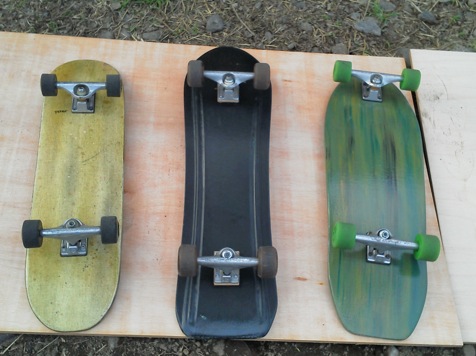The image, taken outside during the day, shows three upside-down skateboards aligned on a long, light tan piece of wood. The bottom piece of wood is juxtaposed with a slightly lighter and broader wooden panel on the right side. The entire setup rests on a surface composed of dark brown soil mixed with dry grass and dirt.

From left to right:

1. The leftmost skateboard is predominantly yellow with black wheels. It has metal bars securing the wheels to the board.
2. The middle skateboard is the longest, spanning the full length of the wooden board beneath it. This skateboard is black with slightly lighter black wheels.
3. The rightmost skateboard is green and appears slightly wider than the other two, though it's about the same length as the yellow one. It features green wheels and some additional details in darker green and black.

All three skateboards add a vibrant contrast to their natural, earthy surroundings.